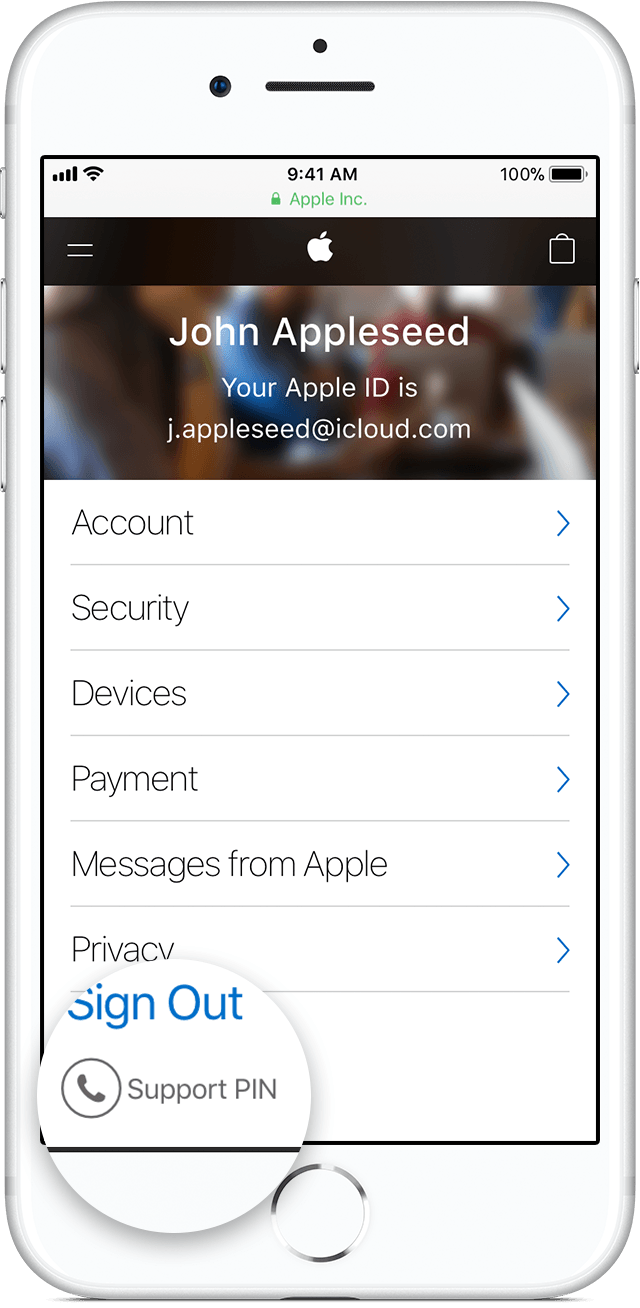In the image, there is a detailed view of an Apple iPhone positioned vertically against a neutral background. The iPhone features a sleek, metallic case that appears to be either white or silver. Notably, the sides of the device include an on-off button and volume controls. The screen of the iPhone displays a wealth of information: it shows the current time as 9:41 a.m., a full Wi-Fi signal, four bars of cellular signal, and a fully charged battery at 100%.

At the top of the screen, there is an Apple logo, followed by the name "Johnny Appleseed." Below this, text displays Johnny’s Apple ID as "j.appleseed@icloud.com." Further down, a list of options is clearly visible, including "Account," "Security," "Devices," "Payment," "Messages from Apple," and "Privacy." At the very bottom of the screen, there is a centrally located round button labeled "Sign Out" and another option for a "Support PIN". The pristine design and organized layout of the iPhone interface are evident from the image, conveying both functionality and aesthetic appeal.